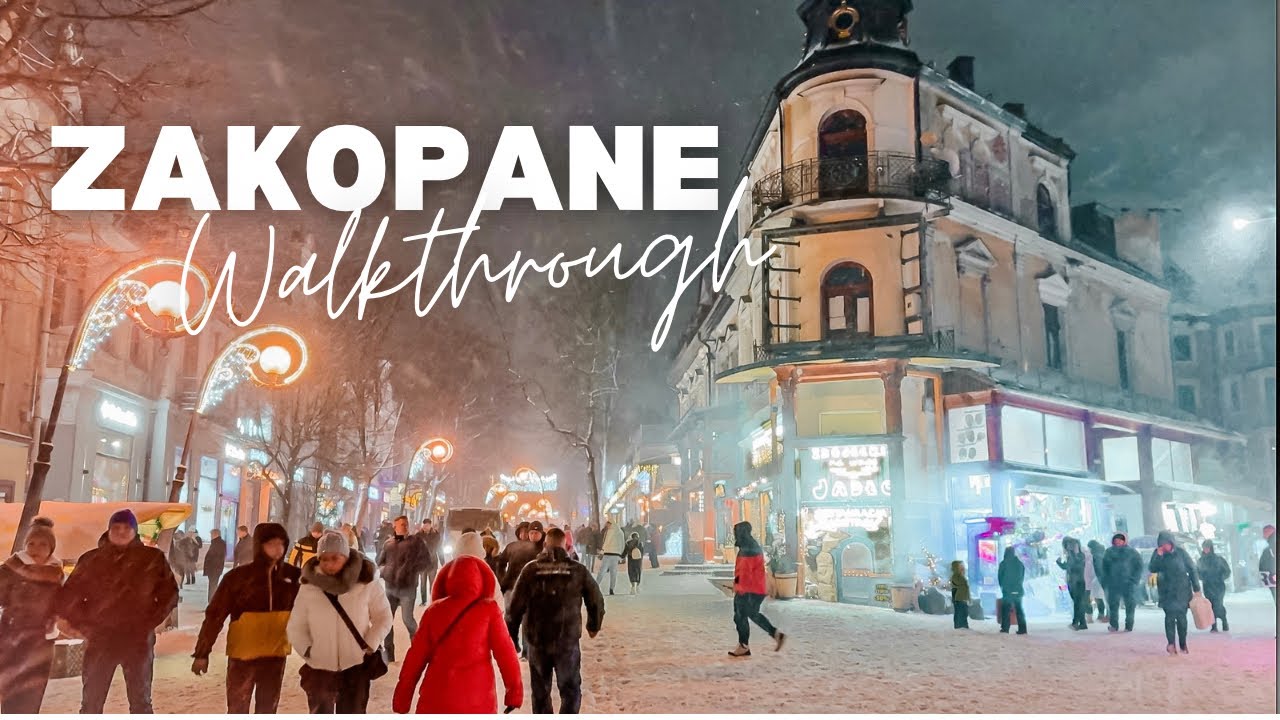The photograph captures a bustling winter evening scene at an intersection in Zakopane, as indicated by the white text in the top left. The streets are filled with people warmly dressed in coats, hats, scarves, and parkas, moving in various directions. Snow blankets the ground, and gentle snowfall adds to the wintry atmosphere. The numerous streetlights, decorated with silver glittering lights and floral-inspired designs, illuminate the scene, offering a fairy-tale ambiance. The buildings along the streets are brightly lit, suggesting a festive or holiday season. Notable is a triangular-shaped building at the corner, featuring three tiers and a yellow façade with black accents, contributing to the lively and vivid street scene. Neon lights add a modern touch to this picturesque winter night in Zakopane.